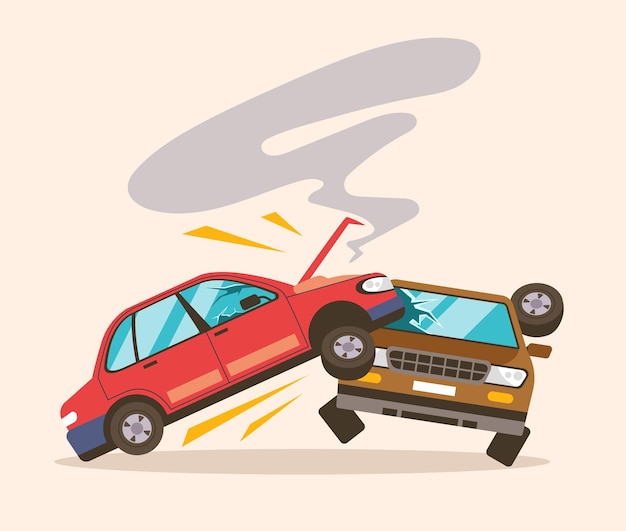The image is a detailed cartoon drawing depicting a collision between two cars against a pale peach background. A red sedan is shown T-boning a brown sedan, with the red car's rear end airborne and its hood open, emitting smoke that forms a large, gray, backward question mark shape pointing into the engine. The brown car, primarily on the ground, has blue glass windows, a wheel that appears to have fallen off, and its remaining wheels are bent and twisted. The scene includes orange lines and yellow triangles accentuating the impact. Both cars cast a circular gray shadow underneath them, indicating the point of collision.